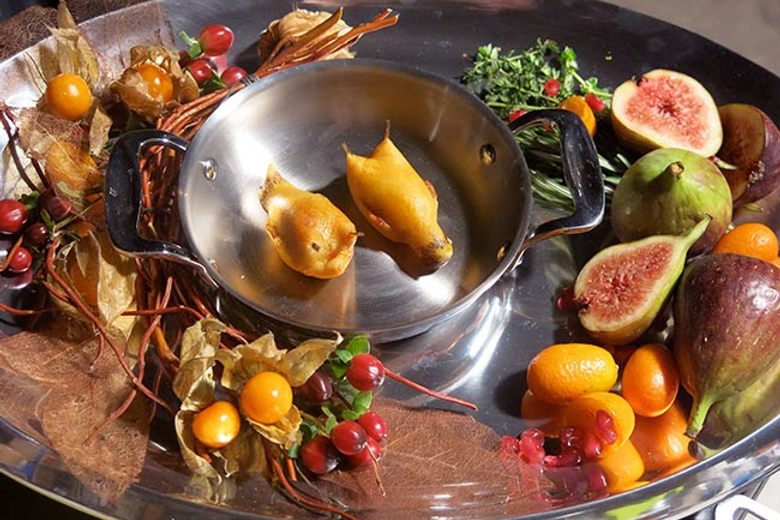A large circular silver platter is filled with an array of colorful fruits, vegetables, and herbs. At the center of the platter is a small, ornate silver bowl with handles, containing two yellow, fried pieces of chiclets. Surrounding the bowl, the platter features a variety of fruits including large orange grapes, small red grapes, figs, persimmons, and small orange citrus fruits. Also present are herbs that resemble basil or cilantro, a few leafy greens, and additional unidentified fruits or berries in shades of purple, pink, yellow, and green. The display is both vibrant and visually appealing, making it a grand and exotic meal offering.